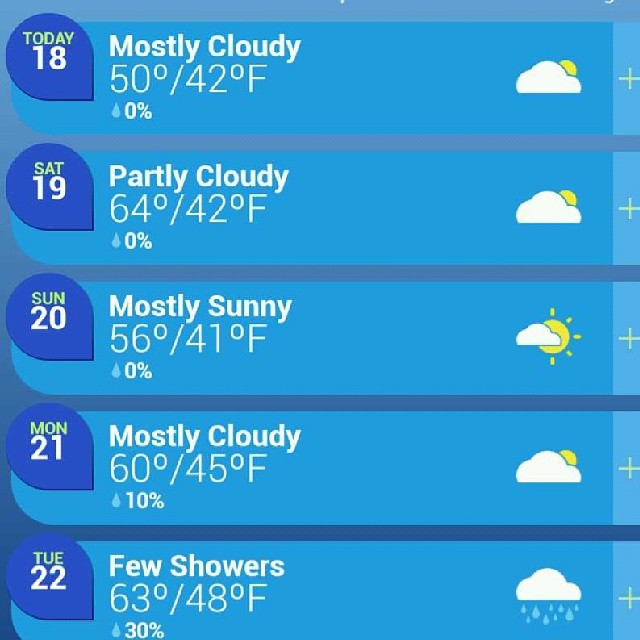This image depicts a 5-day weather forecast chart taken from a digital screen with a blue background and white text. Each day's forecast is represented by a horizontal blue bar that includes the date, weather description, temperature range, and rain percentage. Matching weather icons are displayed on the right side of each entry. 

- **Today, the 18th:** Mostly cloudy with temperatures ranging from 50°F to 42°F and 0% chance of rain.
- **Saturday, the 19th:** Partly cloudy with a high of 64°F and a low of 42°F, 0% chance of rain.
- **Sunday, the 20th:** Mostly sunny, 56°F high and 41°F low, 0% chance of rain.
- **Monday, the 21st:** Mostly cloudy, with temperatures between 60°F and 45°F, 10% chance of rain.
- **Tuesday, the 22nd:** A few showers, with a high of 63°F and a low of 48°F, 30% chance of rain.

There are weather icons next to each forecast description indicating the weather conditions—clouds, sun, or rain. Additionally, there is a small plus sign on the right side of the screen, likely for accessing more detailed information.